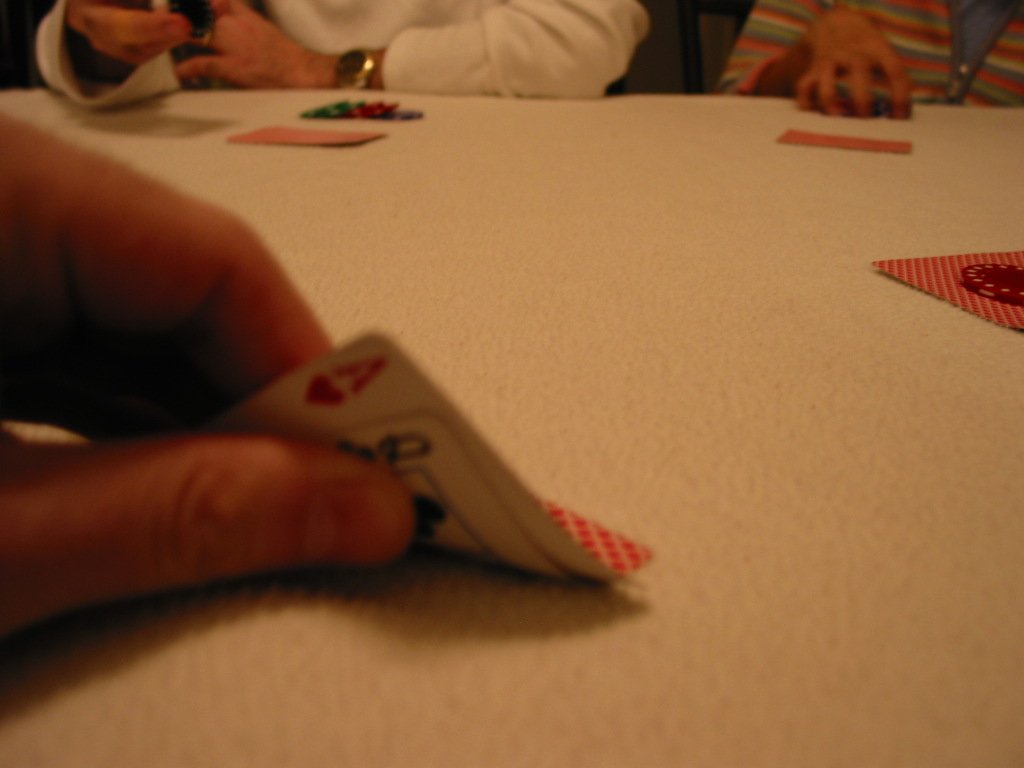In this horizontally oriented image, the setting is a cozy household environment, centered around a table where people are engaged in a card game. The focal point is a hand entering from the left side, displaying a hand of playing cards. The thumb and part of the forefinger are clearly visible, holding the array of cards toward the camera. The foremost card in the hand is the Queen of Clubs, discernible by its partial black club symbol, while just behind it is an Ace of Hearts, slightly out of focus. The scene is bathed in a warm, yellowish-orange light, likely emanating from a nearby kitchen or another indoor light source.

Towards the back of the image, two players are seen seated at the table, each with their cards faced down and a stack of chips in front of them. Adding to the ambiance, a lone card lies in the center of the table on the right side. The overall scene embodies a moment of friendly competition, set in the inviting glow of a home environment.